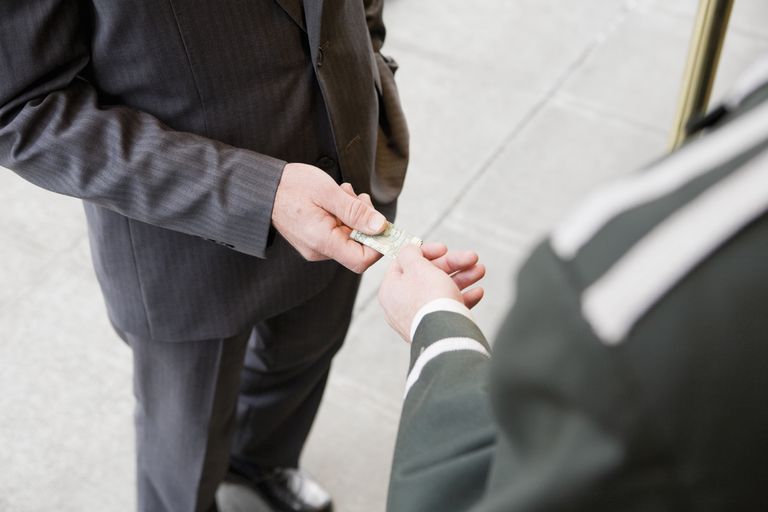In the image, two men are engaged in a transaction, exchanging a folded money bill. The man on the left, dressed in a dark gray suit with a subtle light gray strap pattern, holds one end of the bill. He lacks a tie and wears black or brown dress shoes. The man on the right is clad in a uniform resembling that of a bellboy, featuring a greenish hue with dual stripes on both the shoulder and sleeve. His hand, specifically the left, reaches out to touch the other end of the money bill. Both men's faces are obscured, with the perspective seemingly from behind the man in the uniform, giving the viewer a slightly elevated viewpoint.

The setting appears clean and orderly, with the men standing on what looks like a white tiled surface, potentially concrete, suggesting an outdoor environment possibly near a business, indicated by a gold pillar or bar visible in the upper right corner. The ambient light and the presence of only the two men focus attention on the transaction itself, with no additional text or signage in sight. Both individuals are presumably Caucasian, heightening the neutral tones and textures of the scene.